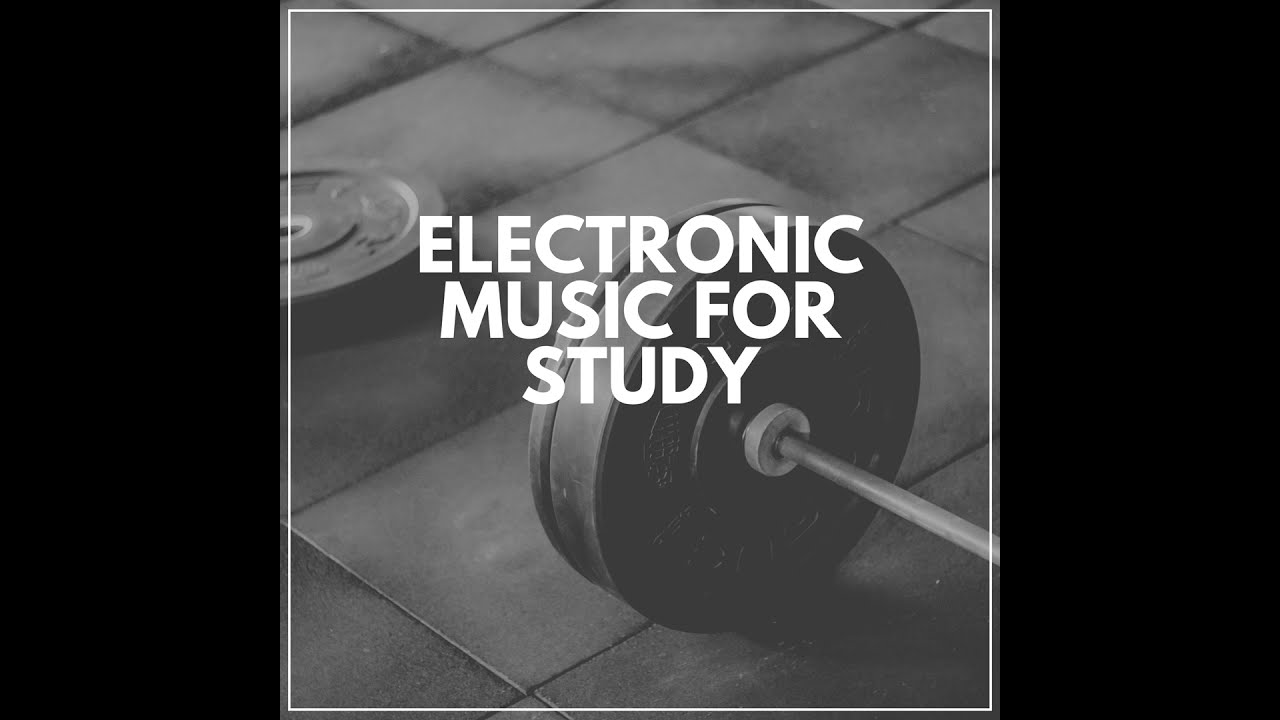The image features a black-and-white, square graphic with a thin white pinstripe border on the inside. The left and right sides have thick black borders, with no header or footer visible. The background showcases a tiled floor that appears to be either concrete slabs or rubber flooring. Centrally, a barbell with weights is seen lying on the ground, with a single, rounded weight plate resting flat in the upper left corner. Superimposed over the barbell, in bold white block letters arranged in three lines, the text "Electronic Music for Study" is prominently displayed, indicating perhaps a YouTube or video thumbnail meant for a study playlist.